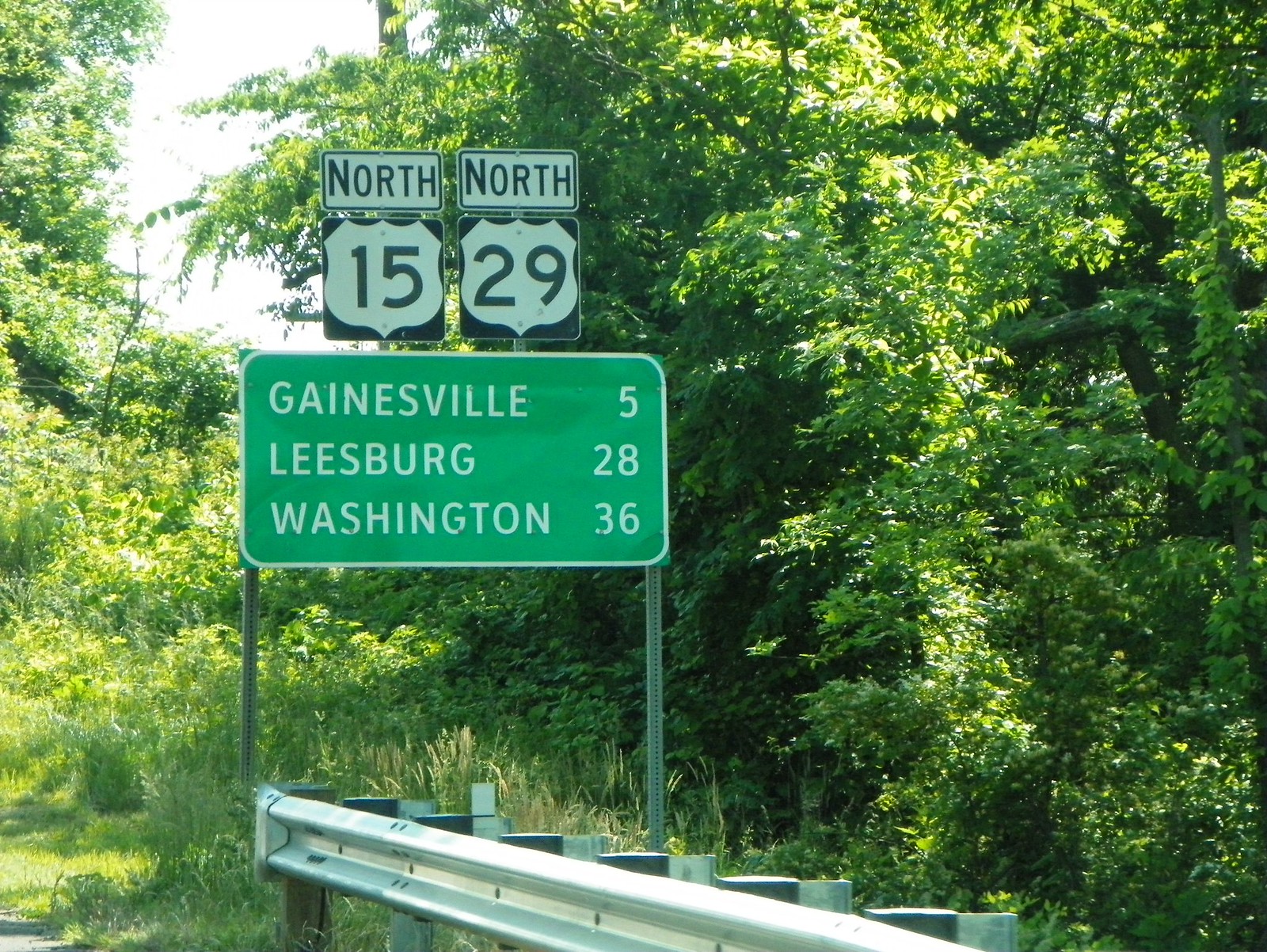In this outdoor photo, there is a dense cluster of thick trees and various bushes, including honeysuckle, with patches of grass and weeds at ground level. A light gray sky is visible through the foliage, casting a gentle glow on the bright green leaves. In the foreground, along what appears to be the side of a highway, there is a silver metal guardrail. Behind the guardrail, a highway sign is held up by two poles. This green rectangular sign has white lettering that indicates distances to various locations: "Gainesville 5, Leesburg 28, Washington 36." Above this sign are two black-and-white shield-shaped signs; the one on the left says "North 15" and the one on the right says "North 29."